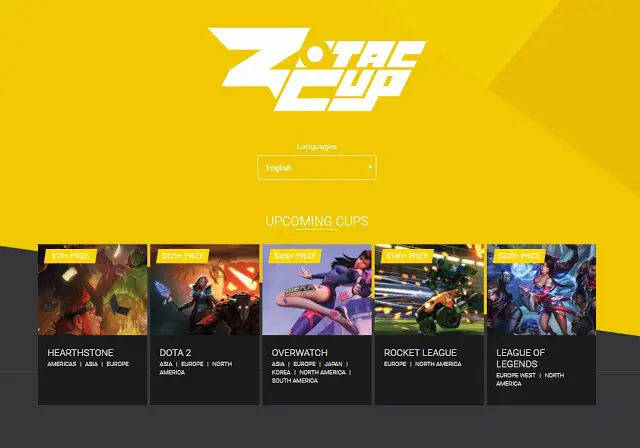The image depicts a website with a predominantly yellow background across the top half. At the very top in white letters, it prominently displays "ZOTAC CUP." Below this title, there is a lightly visible language bar with English pre-selected and a drop-down arrow for more options. 

Underneath the language bar, the text "Upcoming Cups" appears. Below this section, there are five rectangular images representing different gaming tournaments:

1. The first rectangle displays an image featuring a face surrounded by floating objects, labeled "Hearthstone." It lists regions: "America's, Asia, Europe."
2. To the right, there's an image with an orange background showing a person, labeled "Dota 2." It lists the regions: "Asia, Europe, North America."
3. Next, a rectangle shows a female character holding her leg up against a blue background, labeled "Overwatch." This one lists: "Asia, Europe, Japan, Korea, North America, South America."
4. The fourth rectangle portrays what appears to be a car game with white lines in the background, labeled "Rocket League." The regions listed are: "Europe, North America."
5. Finally, an image of a woman with flowing black hair, labeled "League of Legends." It specifies the regions: "Europe West, North America."